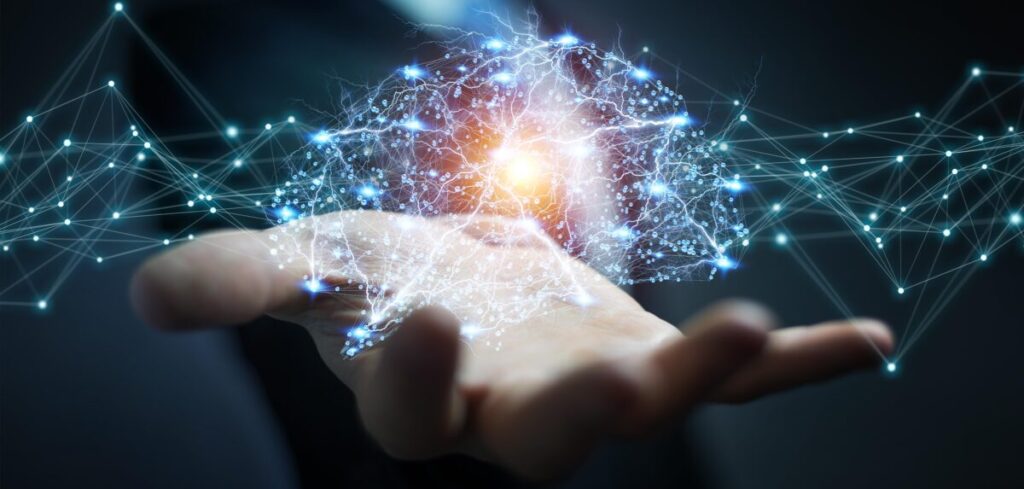The image depicts a digitally enhanced photograph of a white person's hand, palm up, emerging from the top of the frame with the fingertips pointing towards the viewer. Over the palm, there's a striking holographic visualization featuring glowing lines and bright dots, reminiscent of neuronal connections and synapses, giving the appearance of a network of electricity and energy. The central focus, hovering above the hand, is an orb-like cluster of these luminous lines and dots, which resemble a small brain or a condensed sphere of light. Radiating from this central cluster, the connecting lines extend across the image, creating intricate patterns that resemble electronic bars and threads. The overall background is a dark gradient of blue, navy, and black, enhancing the vivid contrast and otherworldly effect of the light and energy emanating from the hand.